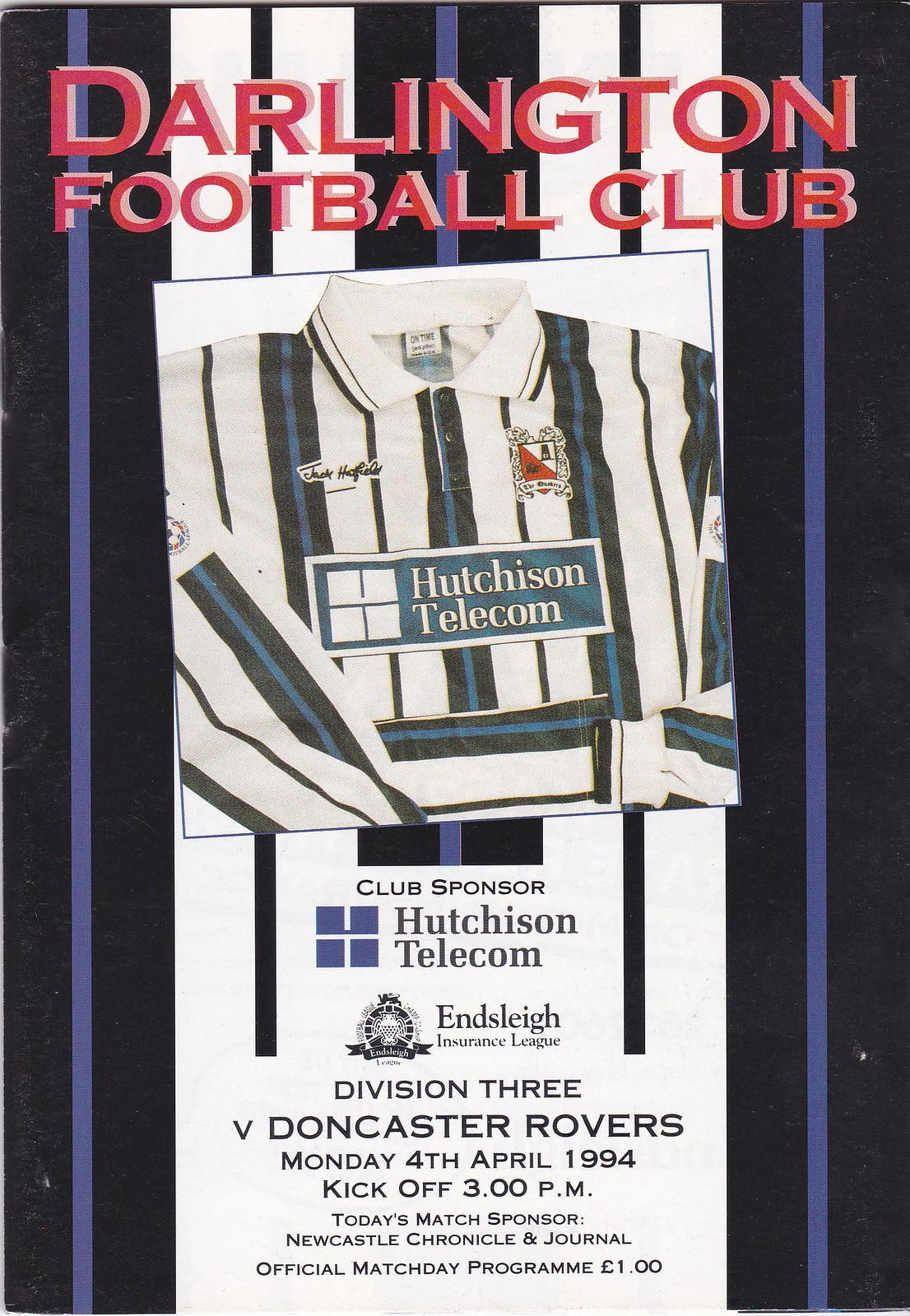This color poster advertises a Darlington Football Club event on Monday, April 4th, 1994, with a kickoff at 3 p.m. Set against a primarily black backdrop with purple and white lines, the top of the poster prominently features "Darlington Football Club" in bold red text with a pink shadow. Central to the design is a photograph of the team's vertically striped jersey, featuring black, blue, and white stripes with "Hutchison Telecom" as the sponsor emblazoned across the chest. Additional text notes the Division III match against Doncaster Rovers, and the sponsorship details mention Hutchison Telecom and Newcastle Chronicle & Journal as the day's match sponsor. The official match day program is priced at 1 euro.